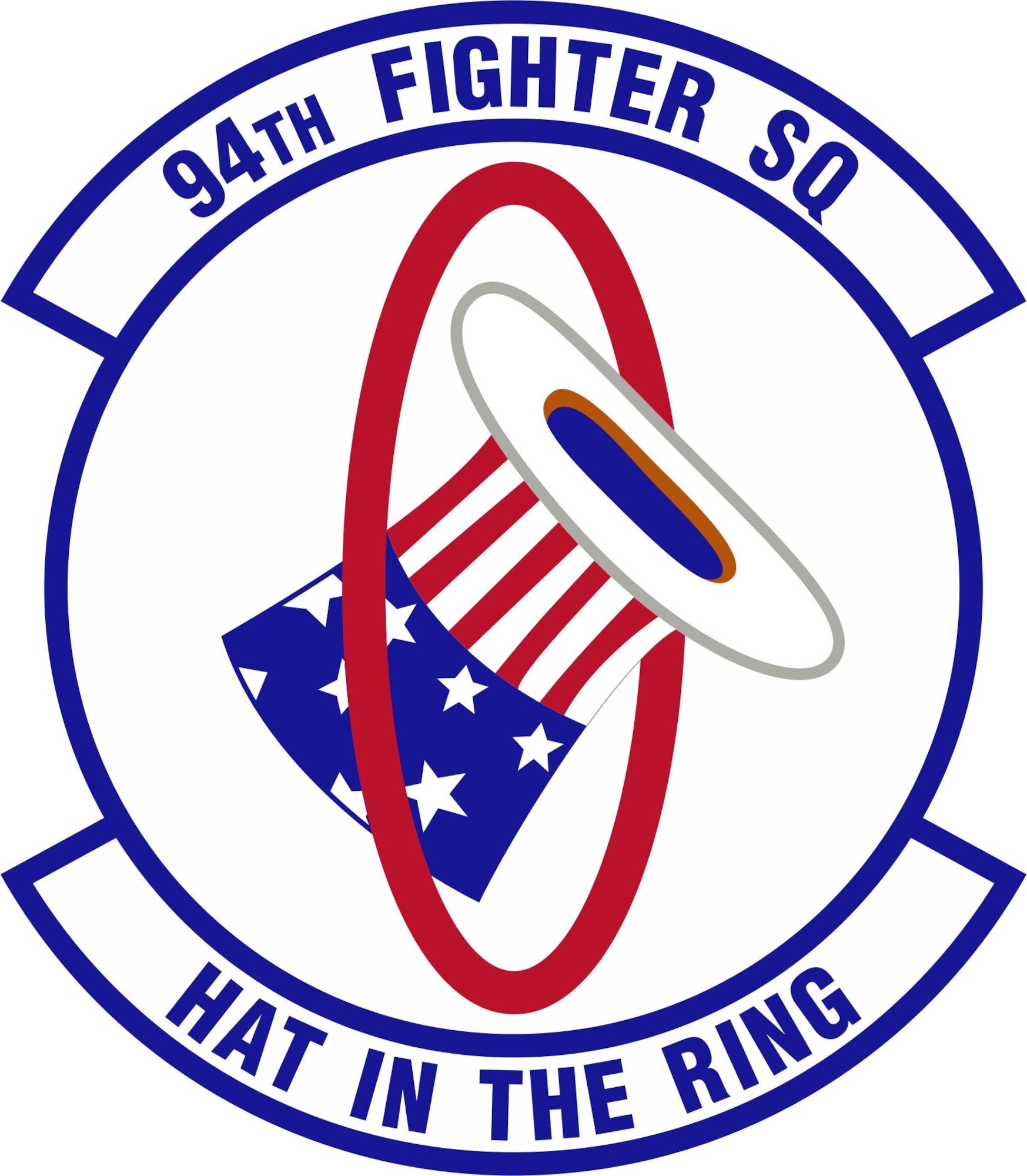The image depicts a vibrant graphic centered on a white background, dominated by the colors red, white, and blue. At its core is a slightly tilted, upside-down Uncle Sam top hat, styled with a blue upper section adorned with white stars, and a lower section featuring red and white vertical stripes. The hat's interior is blue, lined with a gray or silver rim that would typically be hidden if the hat were worn. This hat is artfully balanced at an angle within a thick red ellipse or skinny oval. Surrounding this red oval is a prominent dark blue circle, which itself is encircled by a wider, semi-circular blue banner at both the top and bottom. The top banner reads "94th Fighter SQ" in dark blue capital letters, while the bottom banner declares "Hat in the Ring," also in matching capital letters. This emblematic design is reminiscent of American patriotism, symbolizing elements of the national flag, and adds a whimsical touch to the insignia-style graphic.